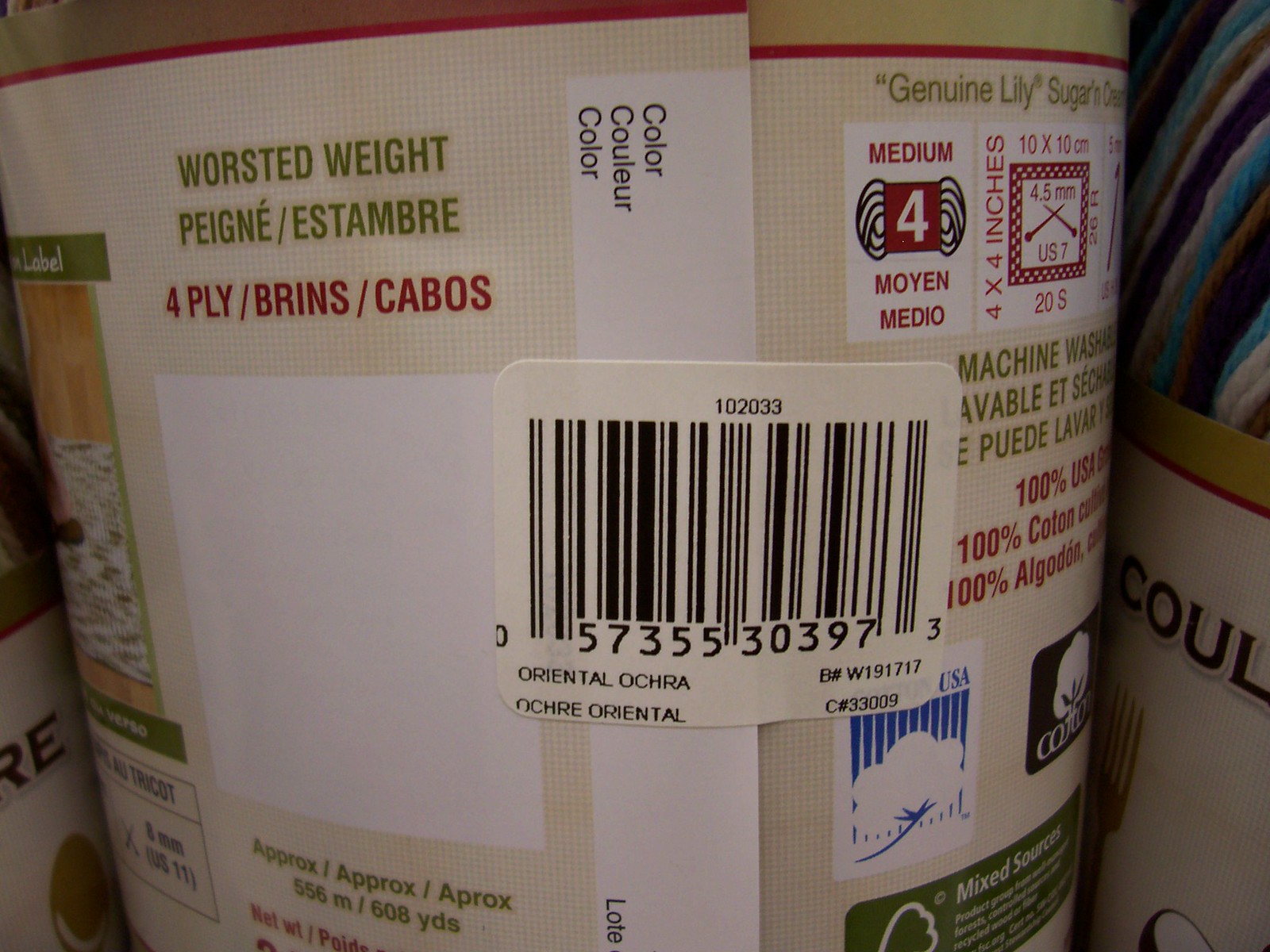A photograph features a tan-labeled packaging item, prominently displaying the word "Worsted" in green font, followed by "weight" in the same green font beneath it. The phrase "four ply" is vividly highlighted in red font below those words. Centrally positioned on the label, there is a white barcode with black stripes and numbers beneath it. Additionally, the label reads "Oriental Okra" in black lettering. 

To the side, several logos decorate the label. The cotton logo, with its black background and white cotton tree illustration, is accompanied by the word "cotton." Another logo, blue and white with the words "Mixed Sources" in white font, features a green tree design. Mention of "608 yards" in green text is visible along with other black and red fonts interspersed on the label. The packaging suggests this might be a type of yarn.